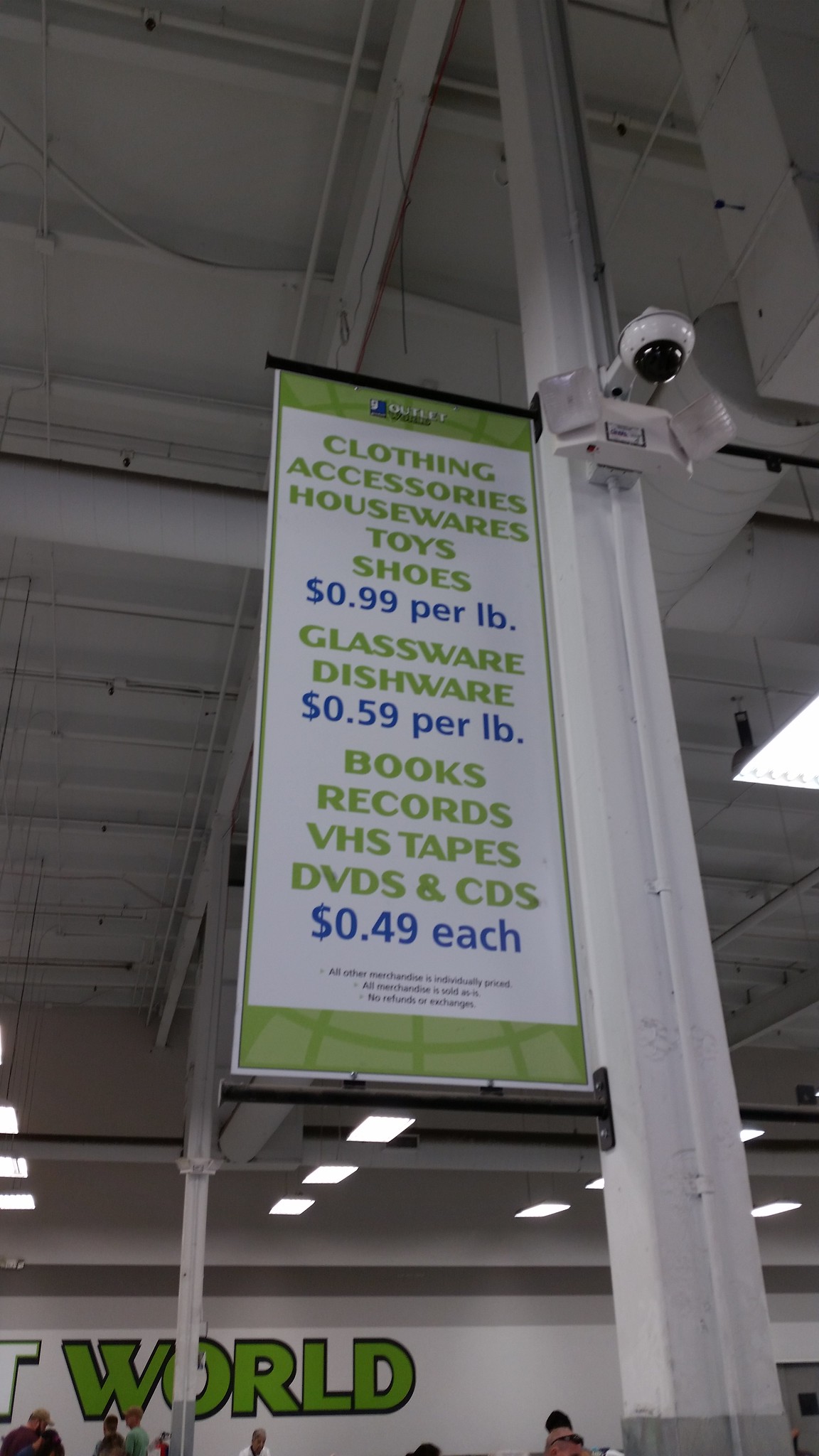This photograph was taken inside a warehouse-style store, capturing a prominent sign mounted on a tall, powder-coated white steel post extending to the ceiling. The post also supports a white security camera with a black lens. The image looks upward, revealing the metallic framework and various exposed utilities, including electrical wiring and plumbing pipes, all painted white. Chains hang from the ceiling, supporting fluorescent light fixtures that illuminate the store.

The sign, secured between black horizontal brackets on the vertical post, features a green border at the top and bottom with a white background in the middle. The text is mainly in green, with some blue accents highlighting the prices. It reads: "Clothing, Accessories, Housewares, Toys, Shoes" on the first line in green, followed by "$0.99 per pound" in blue. The next section lists "Glassware, Dishware" in green, with "$0.59 per pound" in blue below it. The final section advertises "Books, Records, VHS Tapes, DVDs, and CDs" in green, and "$0.49 each" in blue. In the background, the store's back wall is visible, displaying part of a logo with the large green letters "WORLD," partially cut off by the edge of the image. Shoppers can be seen in the distance, their heads just visible beneath the expansive ceiling.